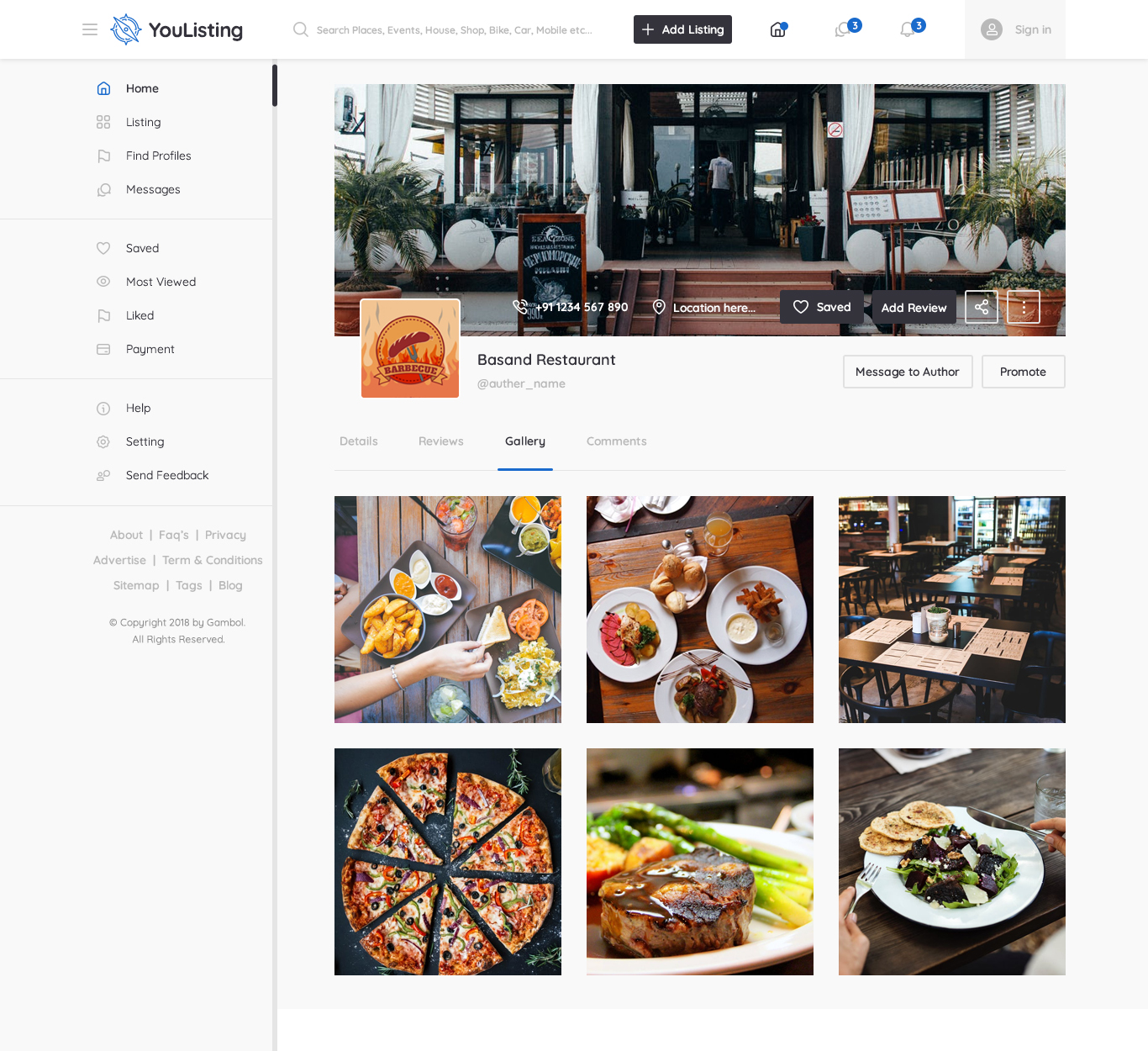The screenshot showcases a listing for "Bassond Restaurant" on the uListing website, where users can add and promote listings. The restaurant's contact phone number is provided as 911-234-567-890. Users can input the restaurant's location, save the listing, and add reviews. The restaurant's icon is a square featuring a blend of orange and peachy colors. There are options to message the author and promote the listing, and the author can be tagged using an "@authorname."

The website menu offers navigation through "Details," "Previews," "Gallery," and "Comments," with the "Gallery" tab currently selected. The gallery displays several food items: one image shows French fries accompanied by multiple dips, a sandwich, and a salad with tomatoes; another features a pizza sliced into triangles with a bite taken out of one piece; a third image presents a salad with round-breaded items; and the final picture depicts the interior of the restaurant with a table set for dining, complete with menus at each place setting.